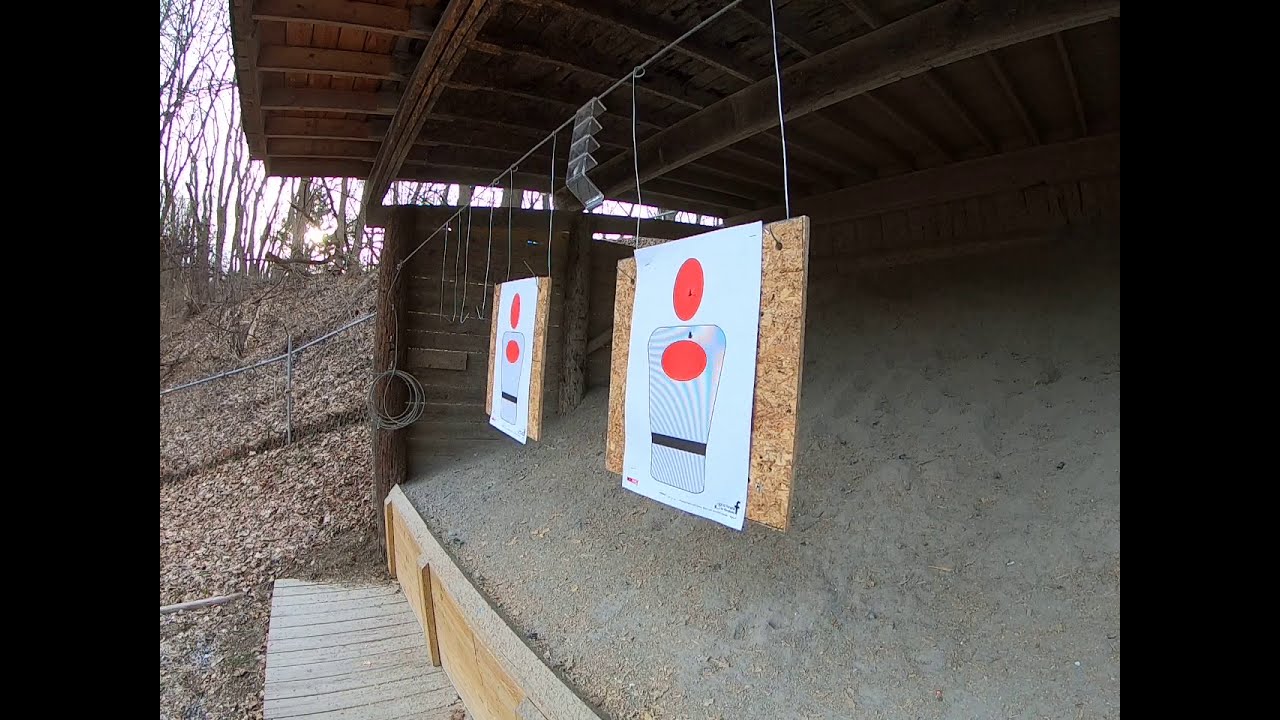In this detailed outdoor image, we see the target area of a shooting range nestled against a hillside covered in fallen leaves and surrounded by bare trees, suggesting it is autumn. The setup features two paper targets, each depicting a human torso with a red oval for the head and another red oval around the chest area. These targets have blue wavy patterns indicating the body shape and a black band at the waist, all printed on white paper. The targets are stapled to square plywood boards, which are suspended by metal wires attached to a horizontal metal wire that traverses from the middle top of the image towards the bottom right.

The plywood boards and targets are part of an open wooden shed-like structure filled with a slanted pile of gray sand, presumably to catch bullets. This structure, approximately in the center of the image, appears to be an open target practice area made out of OSB-type wood with rafters visible. In the background, a chain-link fence runs parallel to the hill, reinforcing the enclosed nature of the shooting range. The image is captured during the daytime, with the lighting suggesting either sunrise or sunset. The overall ambiance is serene yet functional, characteristic of an outdoor shooting range in a natural setting.